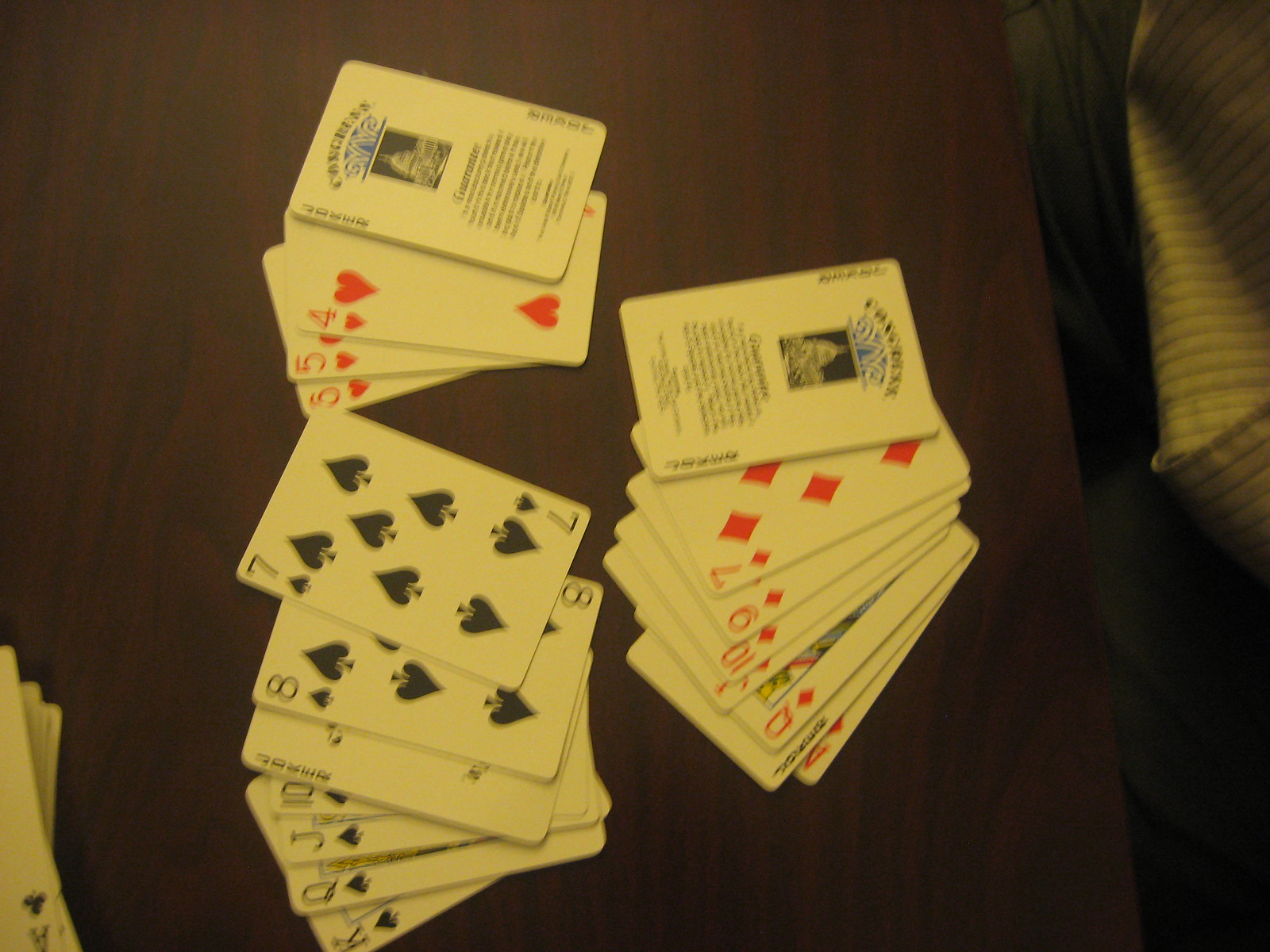A top-down view photograph captures the scene of a card game in progress on a dark stained wooden coffee table. The central focus is on three meticulously arranged sets of cards, indicative of a game like rummy. The first set, positioned towards the bottom left and extending towards the center, features a sequence from the Seven to the King of Spades. Beside it to the right, a joker, played as a wild card, complements a sequence of 3, 4, 5, and 6 of Hearts. Below this set lies another sequence starting from the Six of Diamonds to the Ace of Diamonds, with the joker substituting for the missing Eight of Diamonds.

A chair pulled out to the right suggests recent activity and a player’s presence. The scene hints at an intense moment in the game, where the player has strategically arranged their cards, all neatly in order. The image, rich in detail, draws you into the thoughtfulness and strategy of the card game being played.